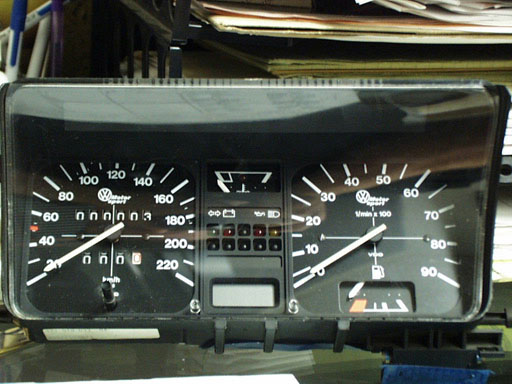The image showcases a Volkswagen speedometer prominently placed on top of a desk, possibly undergoing maintenance. The speedometer on the left displays a range from 20 to 220 and features the iconic Volkswagen logo at its center. The reading on the speedometer indicates three miles. Surrounding the speedometer on the desk, there are various items including stacks of papers and several pins on the left side. The background of the image is filled with additional papers and desk-related objects, contributing to an overall atmosphere of a workspace in a state of active use or repair.